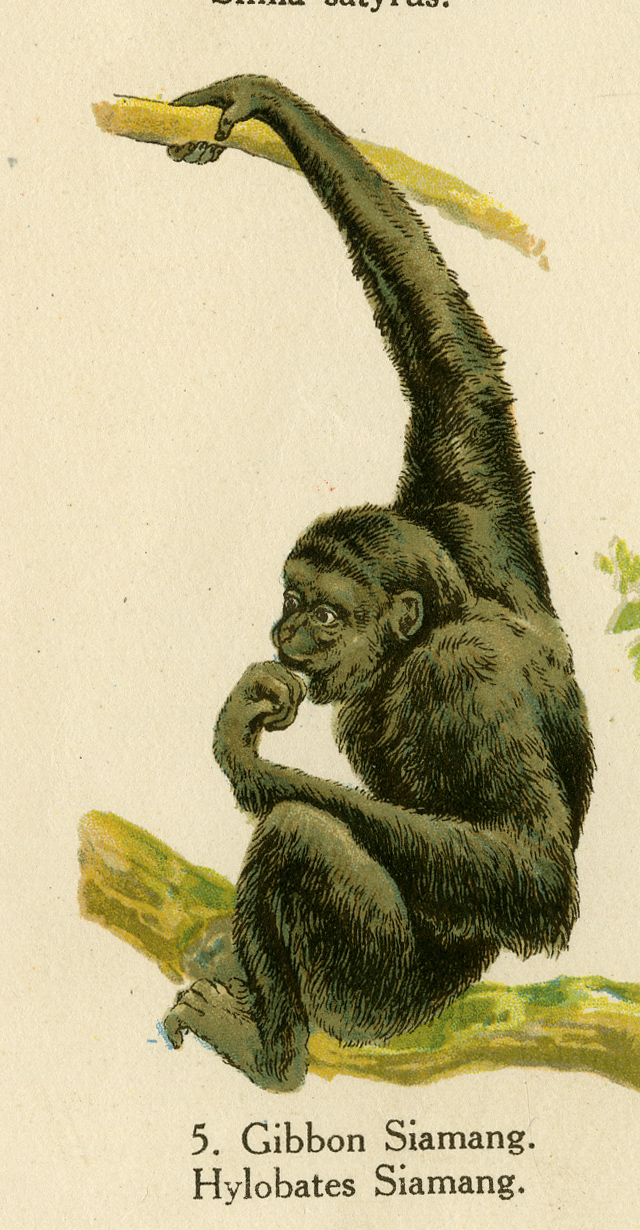This is an old illustrated image depicting a chimpanzee-like monkey, possibly a Siamang given the words at the bottom of the image which read "5, Gibbon, Siamang, Hylobates, Siamang." The monkey is primarily brownish-gray with visible bristles in its fur, featuring hints of bluish tones. It is perched on a branch with its long right arm reaching out to grasp another yellowish branch above, while its other hand is positioned near its mouth, suggesting a thumb or finger close to its lips. The monkey's eyes gaze off to the left, giving it a slightly mischievous expression. Its legs rest on a lower branch and the scene is further detailed with some leaves poking in from the right side. The background of the image is a parchment paper-like tan with little specks, and at the top of the image there are partially visible black words that have been cut off.